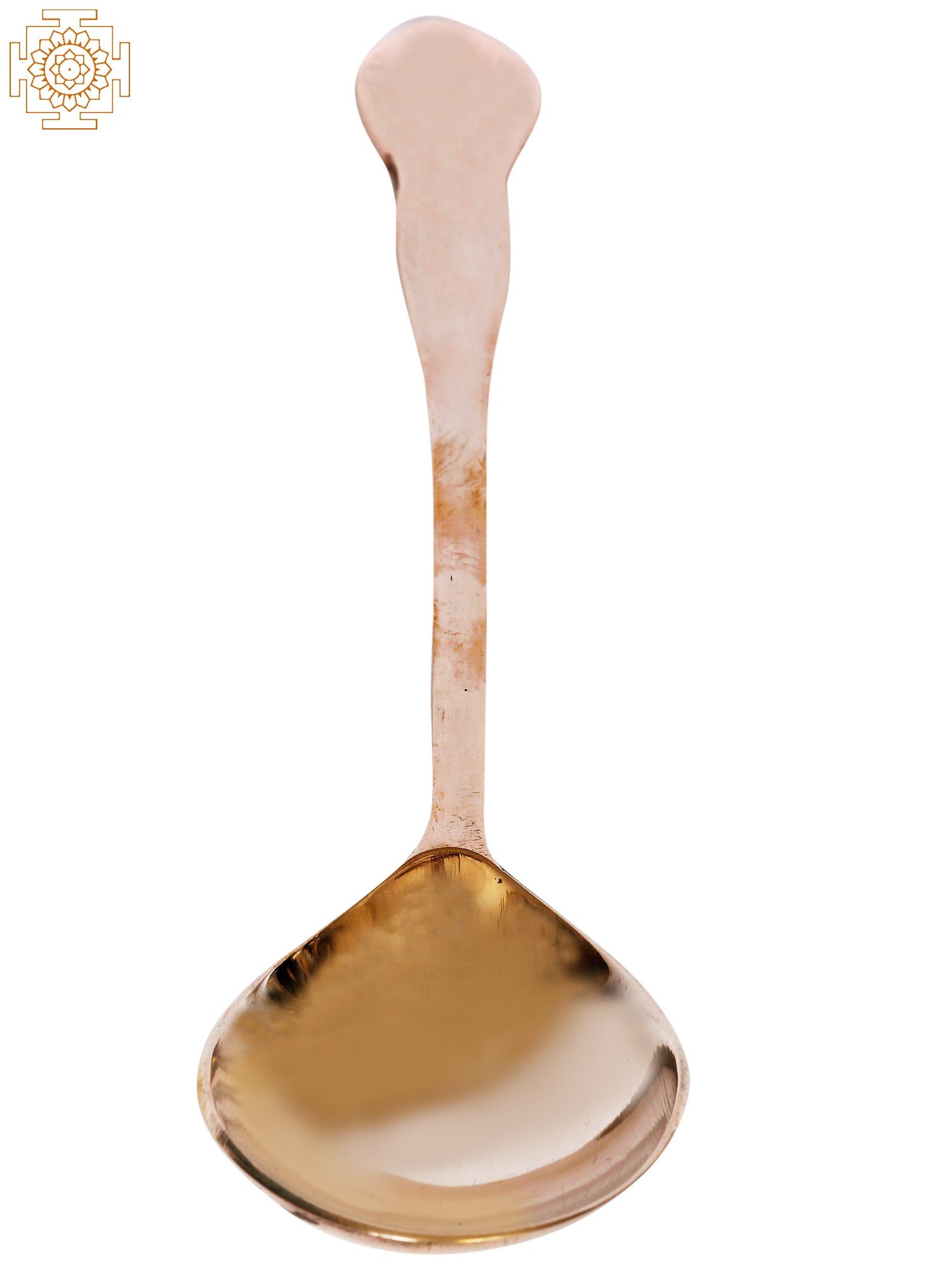The image depicts an undefined brownish object set against a completely white background. Central to this object is a teardrop-shaped, concave surface that closely resembles the bowl of a spoon, containing a reflective, transparent brown liquid that catches and reflects light. This surface seems to show subtle black highlights around its edges. Extending from this bowl is a handle that runs top to bottom; the handle is tinged with an off-white color and shows traces of brown staining. In the top left corner of the image, there is a small, golden logo or symbol. The entire scene lacks any additional background details or context, keeping the focus solely on this ambiguous object and the logo.